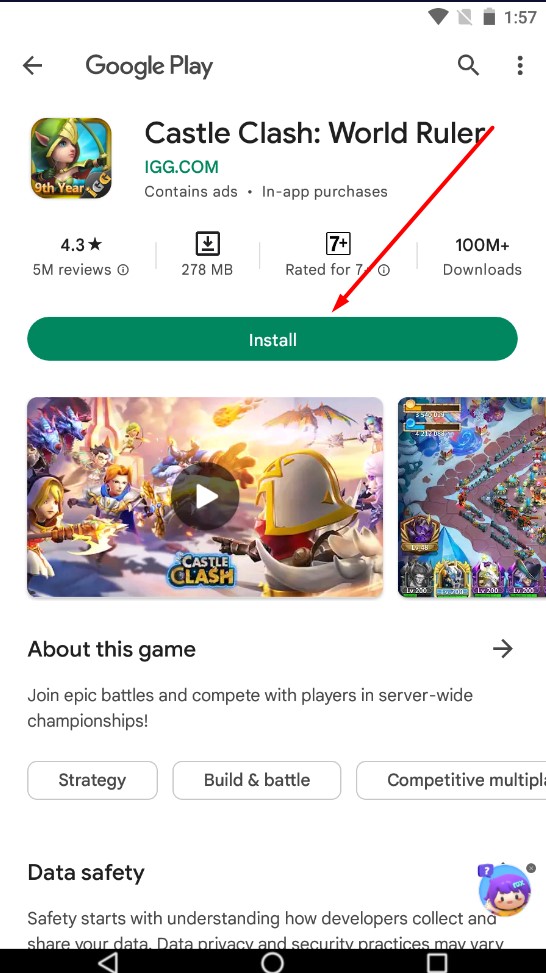The top of the image displays "Google Play" with the time shown as 1:57. Beneath that, it reads "Castle Clash: World Ruler" by IGG.com, with a note that the app contains ads and offers in-app purchases. The app has a rating of 4.3 stars from 5 million reviews and is 278 megabytes in size. A small square icon with the number "7" indicates it's rated for ages 7 and up. The app has over 100 million downloads.

A prominent, large dark green "Install" button is featured, with a thin red arrow pointing at it. Below this section, two screenshots are displayed, one of which appears to be a video related to the game "Castle Clash." 

Further down, there's a description: "Join epic battles and compete in server-wide championships. Strategy, build and battle, competitive, multiplayer." The description transitions into a note about data safety, stating: "Safety starts with understanding how developers collect and share your data."